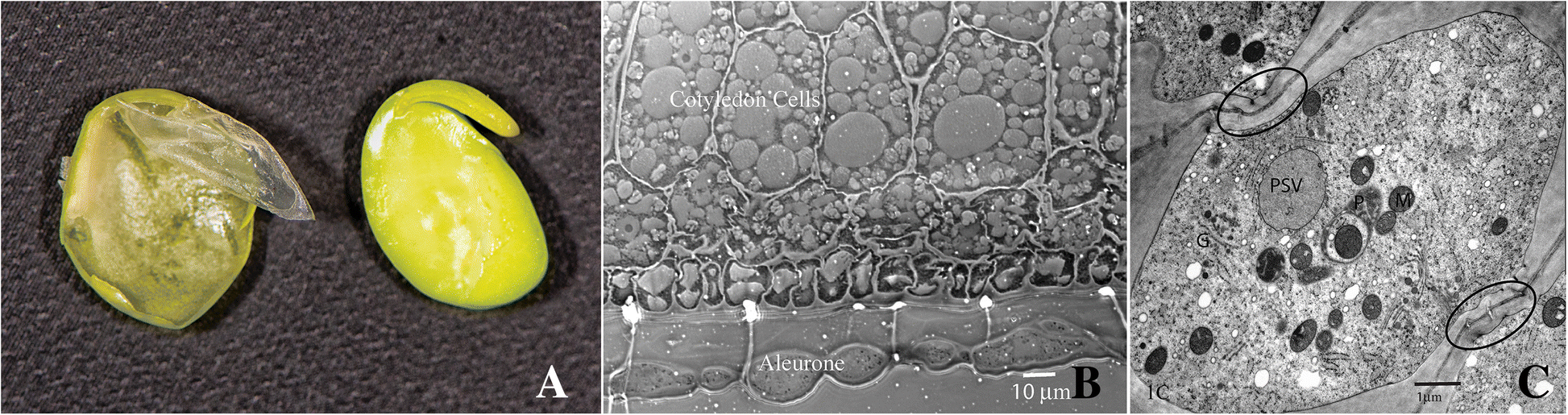The composite image comprises three distinct photos labeled A, B, and C. Photo A, positioned on the left, depicts a seed and a sprouting seedling resting on a dark, possibly fabric, background. The left part of the seedling appears darker and as if its outer skin is peeling off, revealing the fleshy, intact part on the right. Photo B, the central image, is a microscopic, black-and-white view, showcasing cellular structures labeled "collodion cells" with additional annotations "iluron" and "10 μm." Lastly, Photo C, on the right, features another black-and-white microscopic image, showing an oval-shaped cellular structure with circled areas and lines, marked with "PSV" and scattered black dots. All three photos provide a detailed visual journey from a macro view of seeds to intricate cellular details observed under a microscope.